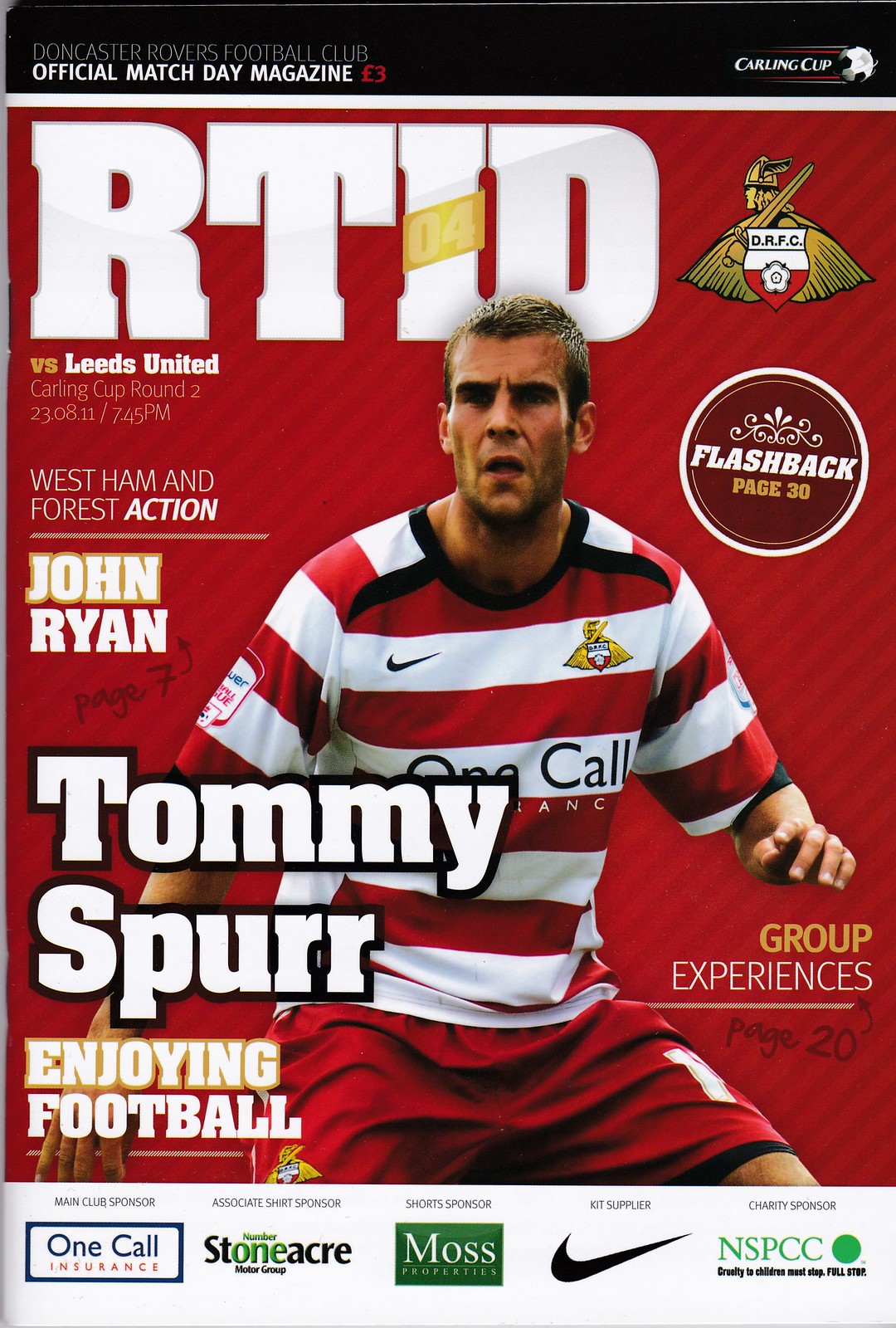This image is the cover of the Doncaster Rovers Football Club's official match day magazine, priced at three euros. The predominant color of the cover is red, featuring diagonal lines in the background. At the top, a black banner announces the magazine's title and price. Below, in bold white letters, it reads "RTID" and "04". The focus of the cover is a photograph of a player, identified as Tommy Spurr, who is wearing a red and white horizontally striped jersey with red shorts. The jersey features a Nike logo, white writing, and a gold design. Information on the cover includes details of a Carling Cup round two match against Leeds United, dated 2011 with a 7:45 PM start time. Additional features mentioned are "West Ham and Forest Action," "John Ryan, page 7," and "Tommy Spurr enjoying football." Sponsors listed at the bottom include Stoneacre, Moss, Nike, and NSPCC.